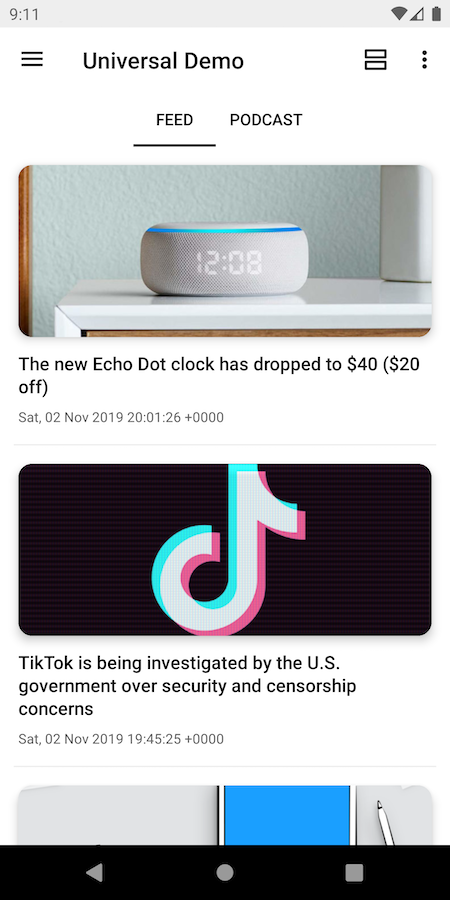Screenshot of a Samsung/Android Phone Interface with News Feed

This screenshot captures the interface of a Samsung or Android phone, clearly distinguished by its unique UI elements. The status bar, located at the top of the screen, indicates the time as 9:11 AM, full Wi-Fi connectivity, a cellular signal strength of about 1 out of 3 or 4 bars, and a fully charged battery. The header displays "Universal Demo" on the left side, with additional settings icons on the right.

Below the status bar, two tab options are visible: Feed and Podcast. The Feed tab is currently active, as indicated by a gray line beneath it. The screen displays two complete news articles and the partial start of a third.

The first article highlights a recent discount on the Echo Dot Clock, now priced at $40, a $20 reduction from its regular price. The accompanying image shows the Echo Dot Clock displaying the time as 12:08, with its white surface and blue light. The article's date is Saturday, November 2, 2019.

The second article reports that TikTok is under investigation by the US government concerning security and censorship issues. This article is also dated Saturday, November 2, 2019, and provides the specific time of publication as 19:45:25 in military time. The image associated with this article features the TikTok logo set against a black rectangular background.

A third article's title begins to appear at the bottom of the screenshot, but it is cut off and not fully readable.